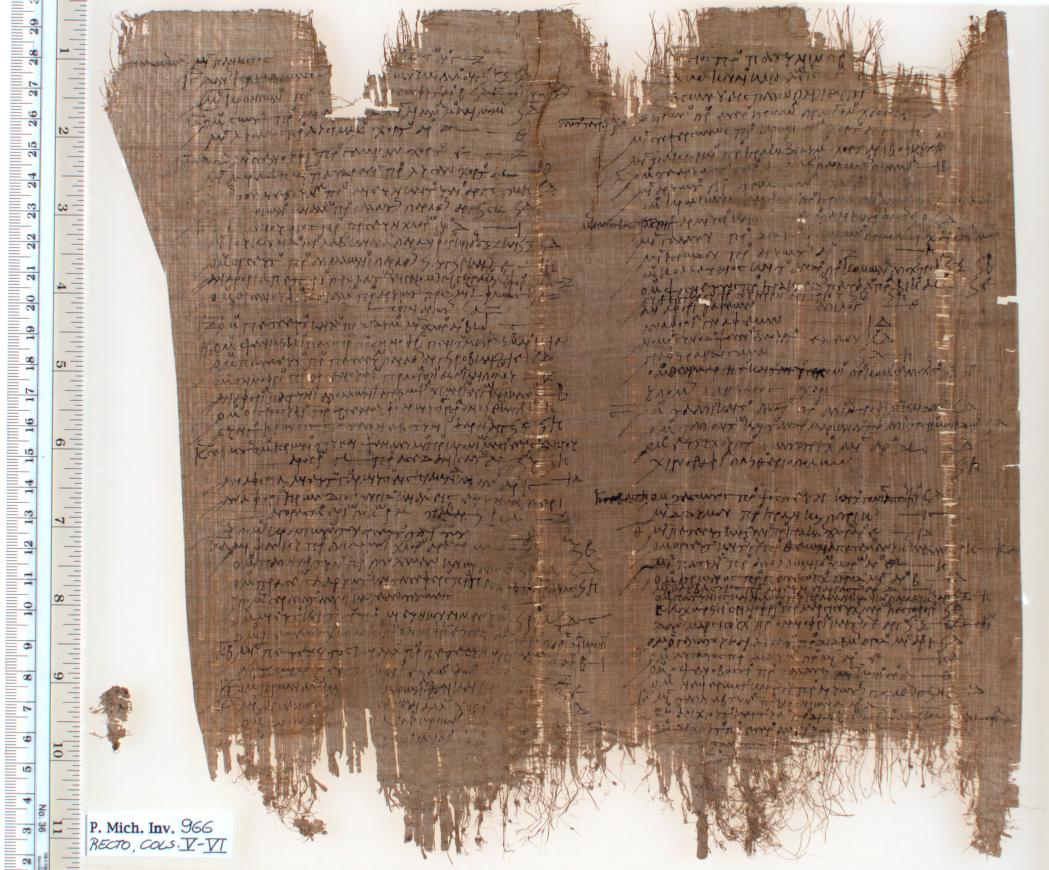The image depicts an ancient scroll or piece of papyrus, appearing to be meticulously preserved and possibly part of a scientific archival process. The artifact, measuring approximately 11 to 12 inches (around 28 to 30 centimeters) as indicated by the measuring tape alongside it, consists of a tan-brown material that might be paper or a fabric-like substance. The writing on the scroll, done in very black ink or paint, stands out vividly against the aged background, suggesting that it has not faded significantly over time. The script appears to be in a foreign language or is too small to decipher. Furthermore, at the bottom left corner of the scroll, in computerized and handwritten text, it reads "PMICN 966. Recto calls 5 to 6" with the latter part inscribed in Roman numerals (V and VI). The edges of the document show signs of fraying, reinforcing its ancient and delicate nature.